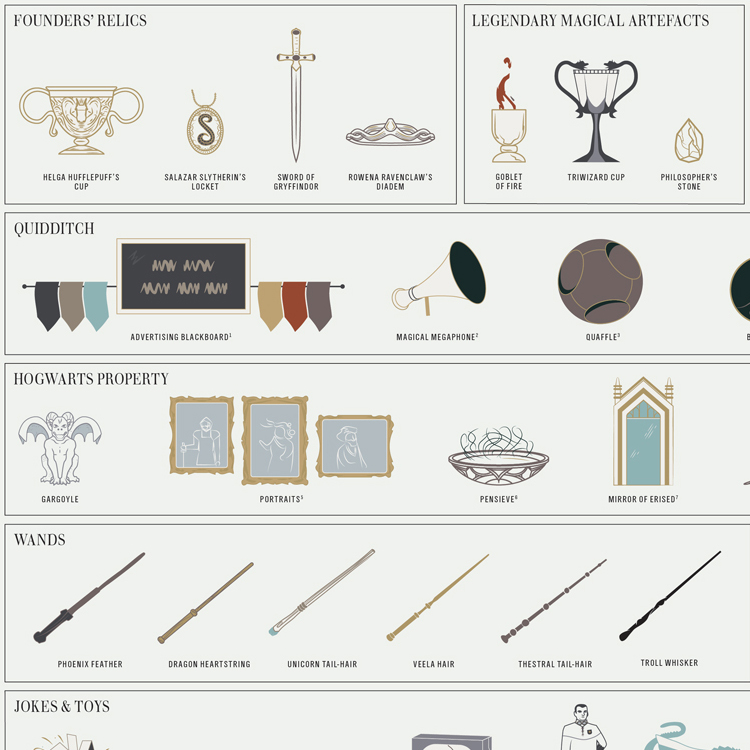The image depicts a detailed, six-section grid of Harry Potter-themed artifacts and items illustrated through digital graphics. The topmost sections are titled "Founder's Relics" and "Legendary Magical Artifacts." The "Founder's Relics" section showcases iconic items such as the Sword of Gryffindor, Helga Hufflepuff's Cup, and Slytherin's Locket. Next to these is the "Legendary Magical Artifacts" section, featuring items like a goblet, the Sorcerer's Stone, and a diadem. Beneath these, the "Quidditch" section includes clipart of flag banners, a megaphone, and a Quidditch ball. The "Hogwarts Property" section displays various objects like statues, framed portraits, a decorative bowl, and a mirror. The next section is dedicated to different styles of wands, listing six in total, each with distinctive names and designs: Troll Whisker, Theatrical Tail-Wearer, Veiler Hair, Unicorn Hair, Dragon Heartstring, and Phoenix Feather. The final section at the bottom is labeled "Jokes and Toys," though it is cut off, preventing the full view of its contents. Overall, there is a distinct digital art style that brings these legendary and magical objects to life.